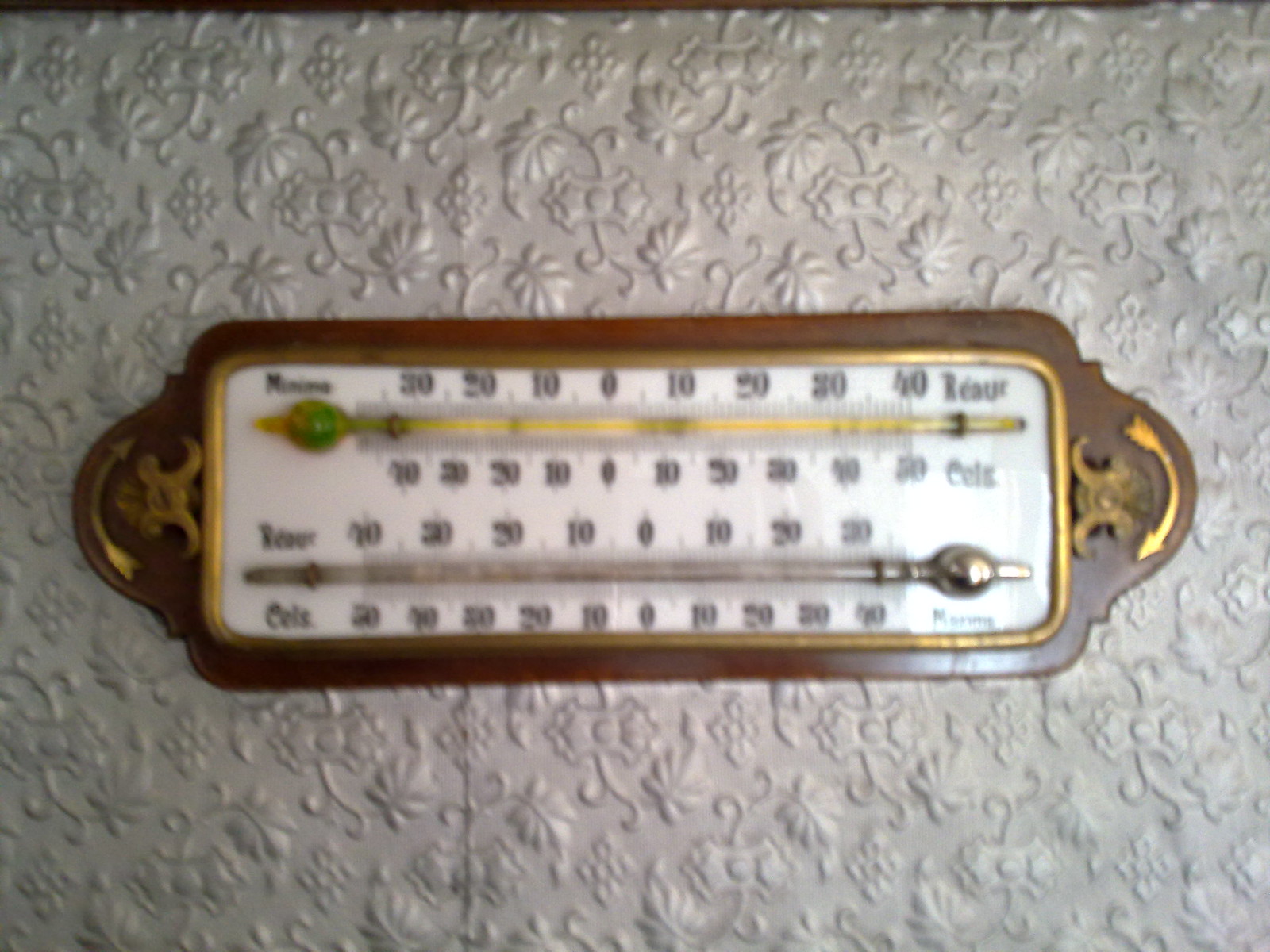The image depicts a vintage thermostat mounted on a dark gray wall adorned with a tactile, raised floral pattern. The thermostat, likely constructed from aged metal, is positioned horizontally from left to right and features a rich, dark brown hue accented with gold trimming. The numerals on the thermostat are elegantly written in a black cursive font. The temperature indicator consists of two parts: the upper component, which has a gold tone with a green tip, and the lower component, which is dark with a silver end. The thermostat's display has a white background, with black numbers stretching from 40 down to 0 in decrements of 10, both above and below the central axis. This artifact exudes an antique charm, resembling items commonly found in antique shops or historic homes.